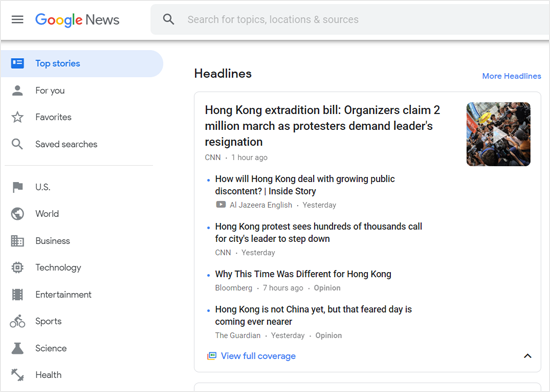This is a detailed screenshot of the Google News homepage. In the top left corner, the page prominently displays the Google News logo, featuring Google's iconic multicolored lettering: a blue "G", followed by red, yellow, blue, green, and then red letters. To the left of the logo, there is a menu button. The word "News" appears in gray next to the logo. Positioned to the right of the logo is a light gray search bar, inviting users to search for specific news topics.

On the left side of the page, there is a vertical sidebar with various icons and corresponding text. This sidebar is organized into two sections, separated by a line divider. The top section contains four items, while the bottom section includes eight. All items are displayed in gray, except for the first item in the top section, which is highlighted in blue. This highlighted item is labeled "Top stories". The sidebar sections are as follows:
- Top Section (highlighted in blue):
  - Top stories
  - For you
  - Favorites
  - Saved searches
- Bottom Section (below the line divider):
  - U.S.
  - World
  - Business
  - Technology
  - Entertainment
  - Sports
  - Science
  - Health

On the right side of the screenshot, the page is titled "Headlines". Within a thin, gray-outlined box, various news headlines are listed. The first headline displayed reads "Hong Kong extraction bill".

This comprehensive layout ensures that users can easily navigate through different categories and access the latest news updates efficiently.